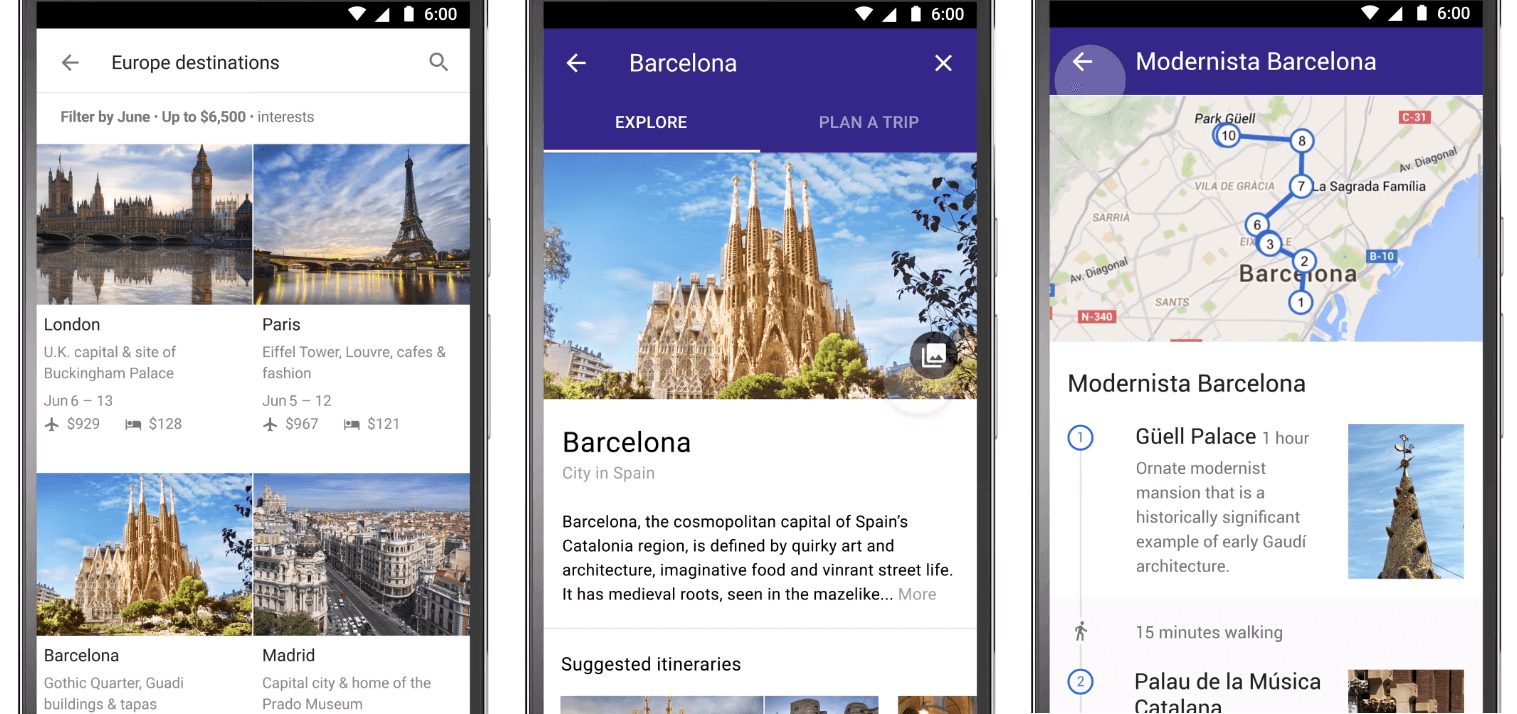---

**Explore Iconic Destinations: A Journey Through Europe**

*Left-side visuals of the image:*

- **Navigation Elements:** The far left of the image displays various icons including destinations, a left arrow, and a magnifying glass for search functions.
- **Metrics Highlight:** By June, the count reaches up to 6500, showcasing growing interest.

*Central visuals capturing London:*

- **Illuminated Skyline:** The lights illuminate London's iconic buildings against a tranquil, blue sky dotted with quiet clouds.
- **Waterscape:** Reflective waters mirror the cityscape, enhancing the serene beauty of the UK capital.

*Parisian Attractions:*

- **Date Specifics: June 6th:** Time marking at 13:929, with financial metrics indicating a value of 128 dollars.
- **Iconic Structures:** The skyline features notable architectures like the Eiffel Tower and the Louvre, famed for their historical and cultural significance.
- **City Atmosphere:** Balmy skies and reflective waters set the scene for the Parisian ambience.
- **Cultural Hub:** Renowned cafes and the fashion district are highlighted.

*Spanish Highlights:*

- **Financial Indicators: June 5th:** With a recorded value of 12,967 dollars and 121 dollars, reflecting some economic aspects.
- **Barcelona:**
    - **Visual Representation:** Showcases the city within the context of Spain, including the Gothic Quarter known for its historic buildings and tapas culture.
    - **Cultural Icons:** Features notable landmarks including a tall building amid classical architecture with references to modern icons.
- **Madrid:**
    - **Urban Life:** Depicts Spain’s capital city, home to the esteemed Prado Museum and diverse urban life.
    - **Color Palette:** Vivid depictions using shades of blue, enhancing the city’s captivating beauty.

*Around Europe:*

- **Sarajevo:**
    - **Regional Flavor:** An artistic narration of Sarajevo’s vibrant street life, nuanced with eclectic art and architectural styles.
- **Madrid and Barcelona Mapping:** Top right shows specific insights of Madrid and Barcelona, adding layers to the historical and cultural context.

- **Gale Palace:** A significant ornate modernist mansion featured for its historical importance, with a final note excluding Burlington from this context.

*General Context:* The entire visual narrative interlinks with historical markers, cultural highlights, economic metrics, and iconic landmarks, painting a detailed exploration of Europe’s most beloved cities.

---